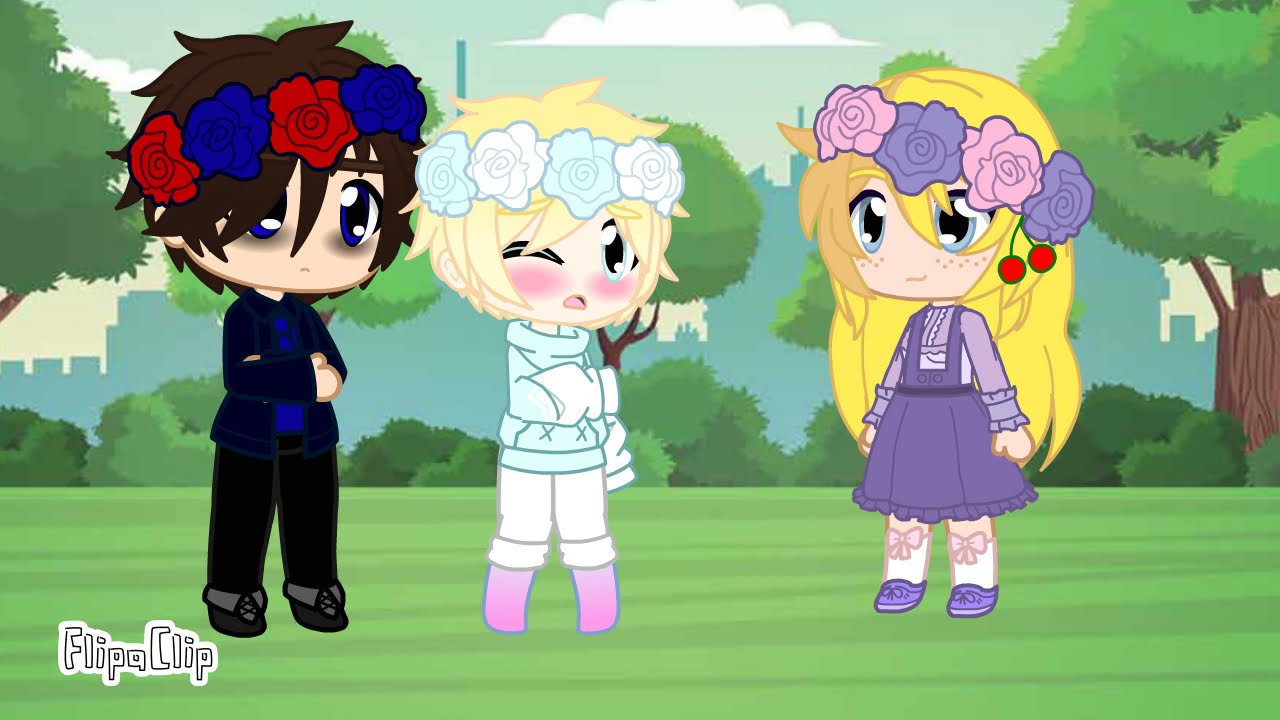In this animated image set in a park-like environment, three cartoon characters stand prominently in the center on a flat grassy field adorned with green bushes. The sky is a blend of bluish and greenish hues with scattered clouds, and you can see a silhouette of a castle with stone walls in the background.

On the left stands a male figure with a large head, big blue eyes, a small mouth, and spiky brown hair adorned with blue and red flowers. He is dressed in black clothing, with arms crossed confidently.

In the middle is a female character with spiky short blonde hair, complemented by turquoise and white flowers in her hair. She has dark eyes, a small mouth, rosy cheeks, and is dressed in a turquoise sweater, white rolled-up jeans, and pink shoes.

On the right is another female figure with long blonde hair, decorated with pink and purple flowers and a cherry. She has big eyes, freckles, and wears a purple dress with matching purple shoes.

The digitally created scene, titled 'Flip a Clip' as indicated by the text in the bottom left corner, uses a vibrant color palette featuring shades of green, blue, red, pink, and purple. The overall style resembles a whimsical cartoon, suitable for a younger audience.